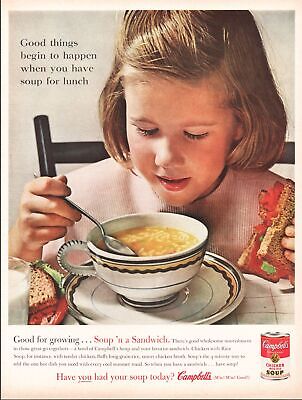This vintage Campbell's Soup advertisement, likely taken from a colorful print magazine or newspaper, features a young girl enjoying a wholesome lunch. The ad is framed by a white border, which is wider at the bottom and houses multiple lines of text, albeit some of it blurry. The vibrant central photograph shows the girl seated in a dark brown wooden chair as she looks down, focused on dipping a silver spoon into a teacup filled with tan-colored soup brimming with white noodles. The teacup, made of white porcelain, sits elegantly on a matching round saucer. She's also holding a tomato-filled sandwich in her left hand, reinforcing the text on the top left of the image: "Good things begin to happen when you have soup for lunch." A glass of milk is placed at the bottom left corner of the table. The ad’s background has a subtle pink hue, and at the very bottom-right corner, a can of Campbell's Chicken Noodle Soup is displayed, accompanied by the phrase, "Have you had your soup today? Campbell's." The overall scene is well-lit and inviting, underscoring the nourishing and comforting essence of having soup for lunch.